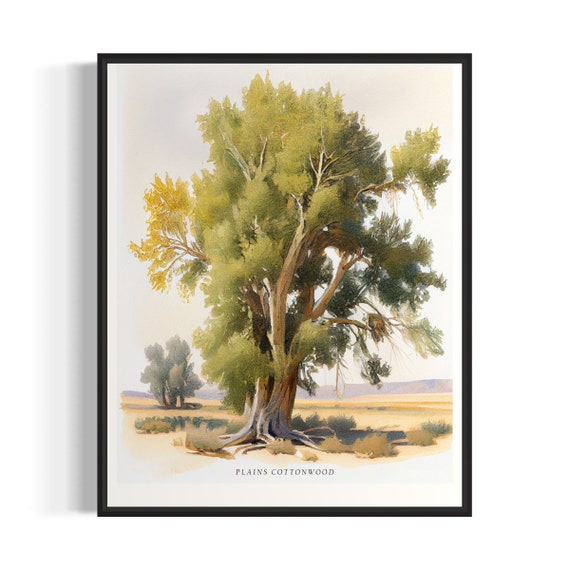This semi-realistic painting, titled "Plains Cottonwood" as indicated by the black text at the bottom, is depicted on a white canvas within a thin black frame that casts a slight shadow. The focal point is a large, mature cottonwood tree with a broad, dusty grayish-brown trunk that splits into four or five main branches, giving rise to numerous smaller branches. The tree is set against an arid landscape of yellow, desert-like dirt with patches of olive-toned grass. The leaves are primarily light green on the left side, transitioning to darker green and a few yellowish hues on the right, creating a shaded effect under the sun. Visible roots add to the ancient appearance of the tree. In the background, another cottonwood tree stands amongst foothills, with purplish mountains faintly outlined in the distance. The overall impression of the painting is one of an old, weathered tree standing resilient in a dry, plains region.